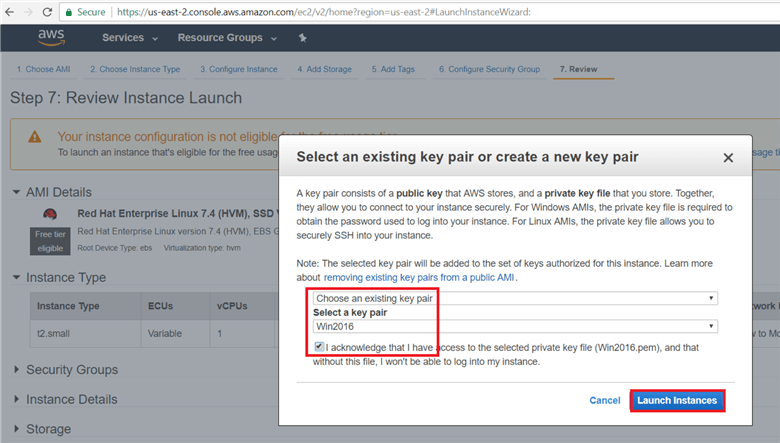**Detailed Caption:**

The image depicts a detailed screenshot of an AWS (Amazon Web Services) console web page, identifiable by the URL starting with "https://console.aws.amazon.com" and the familiar Amazon branding featuring the smiley face. The main interface, rectangular in shape, is partly obscured by an overlay indicating interaction with a secondary window.

The underlying page, partially visible and slightly greyed out, appears to be the main AWS management console with a prominent search box at the top. Below the URL bar, two dropdown menus are labeled "Services" and "Resource Groups," positioned on the left side.

The overlaying window, marked for enhanced clarity, displays content relating to the configuration of an EC2 instance. At the top, it mentions "Step 7: Review" with a warning highlighted in yellow stating that the instance configuration is not eligible, accompanied by more detailed instructions underneath.

A distinct section within this overlay window focuses on key pair options, labeled "Select an existing key pair or create a new key pair." This section is encased in a red rectangular border for emphasis. Within this red box, a dropdown menu allows the user to "Choose an existing key pair," currently set to "WIN2016," which is also selected via a radio button. 

At the bottom of the overlay window, another red rectangular box highlights the "Launch Instances" button, ready to be activated to proceed with the instance deployment.